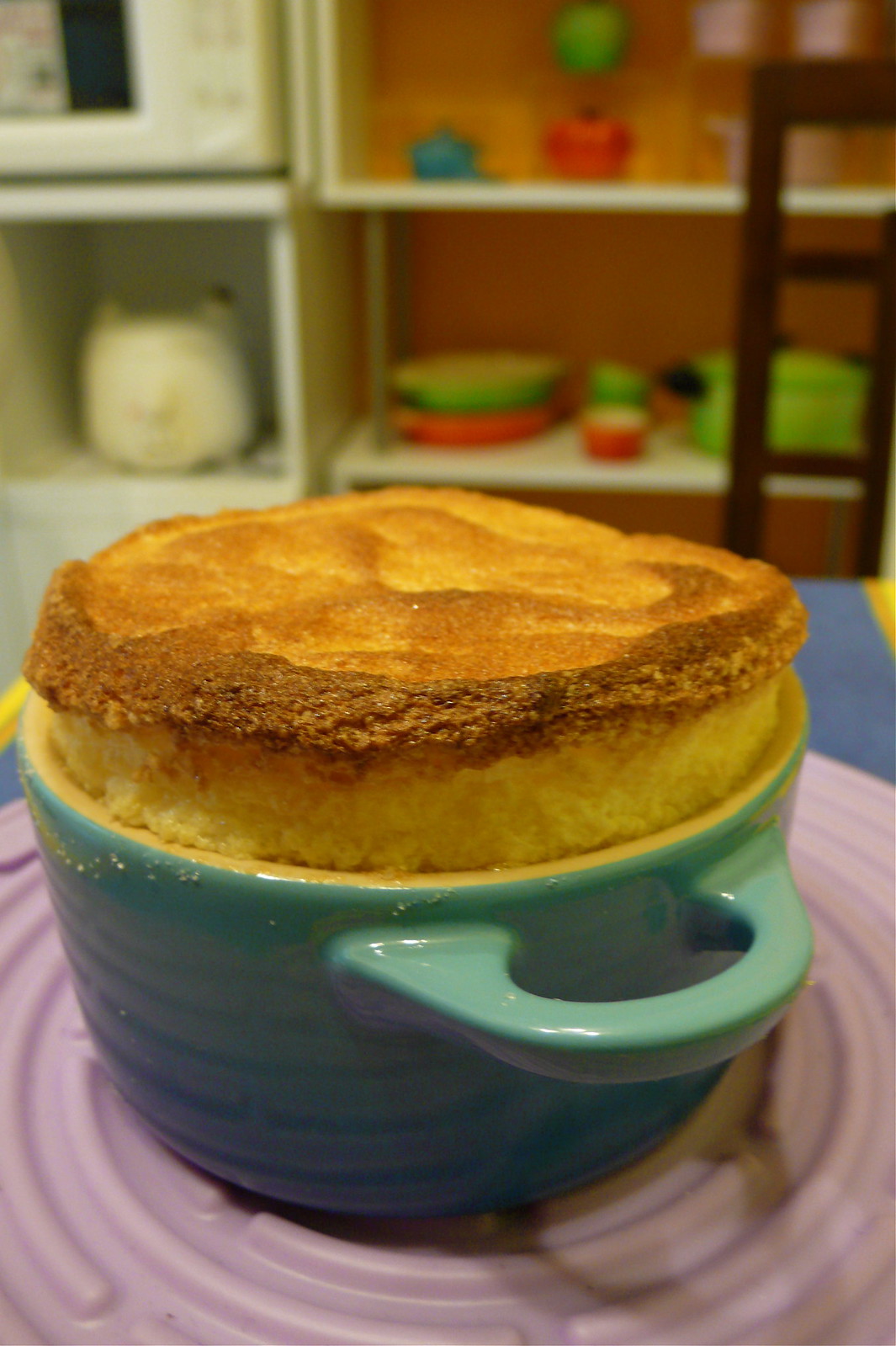In this detailed color photograph, the focal point is a beautifully puffed vanilla souffle, baked to a light golden perfection with a darker golden brown crust on top. The souffle is elegantly presented in an aqua-colored ceramic crock, complete with a handle on the right side, rising about an inch above the dish's rim. This ceramic crock sits on a light lavender-colored plate atop a blue counter, adding a subtle pop of color to the composition. The background reveals a cluttered kitchen scene with white shelves housing a variety of kitchen items, including a rice cooker, microwave, and assorted casserole dishes and cookware. The overall image captures a moment of culinary craftsmanship within a realistic, representational style.